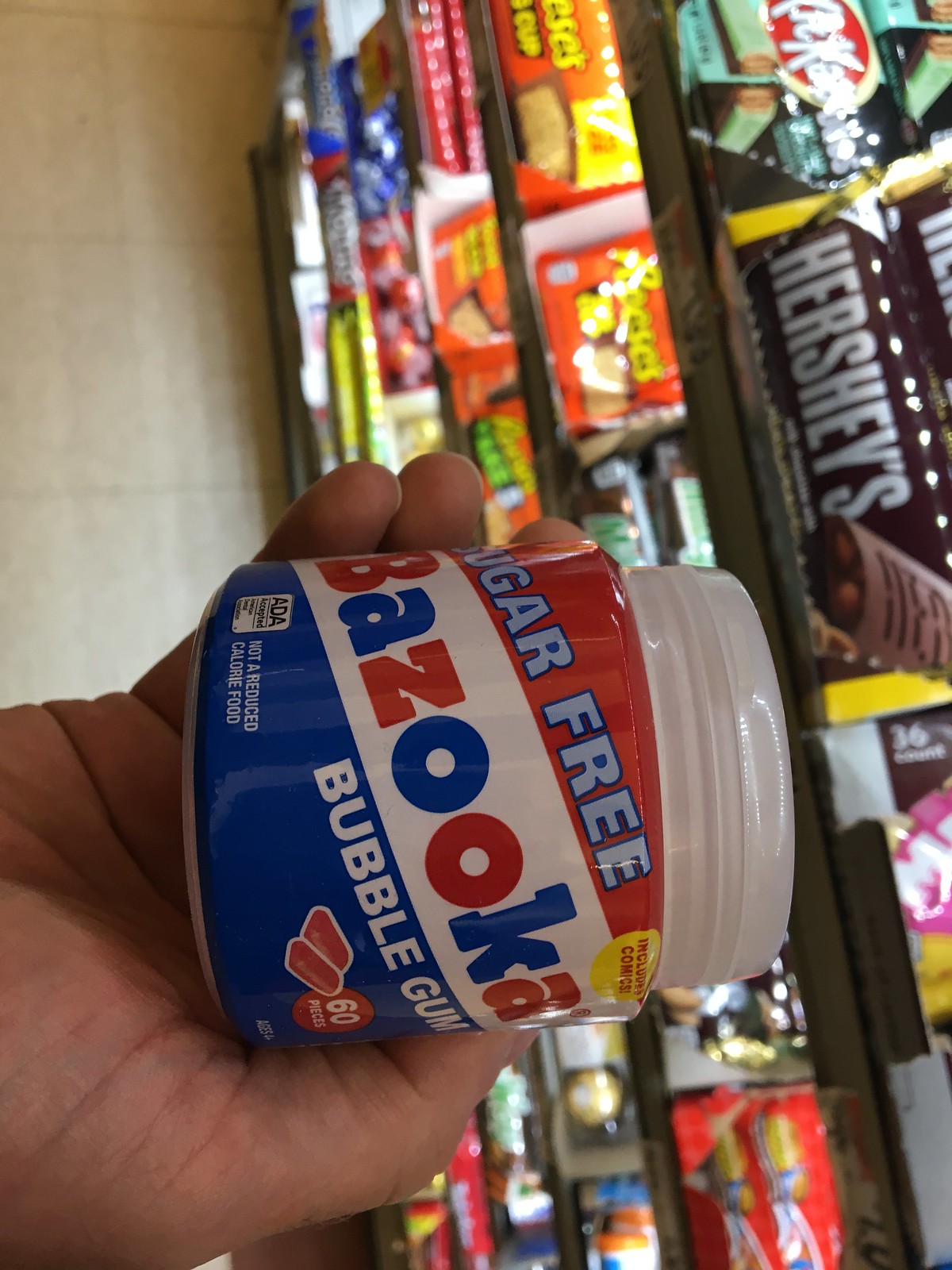In this sideways image, a person is holding a canister of Bazooka bubble gum in the candy aisle of a convenience store. The canister has a white top and a red, white, and blue label with diagonal stripes. The text reads "Sugar-Free" on the red stripe, "Bazooka" in alternating red and blue letters on the white stripe, and "Bubble Gum" on the blue stripe. It also mentions "Includes Comics" on the top right and "60 pieces" on the bottom. The man is holding the canister in his right hand, with his palm and two fingers visible in the bottom left corner of the image. The background is filled with various chocolate bars like Hershey's, Kit Kats, and Reese's, emphasizing the setting of a store.